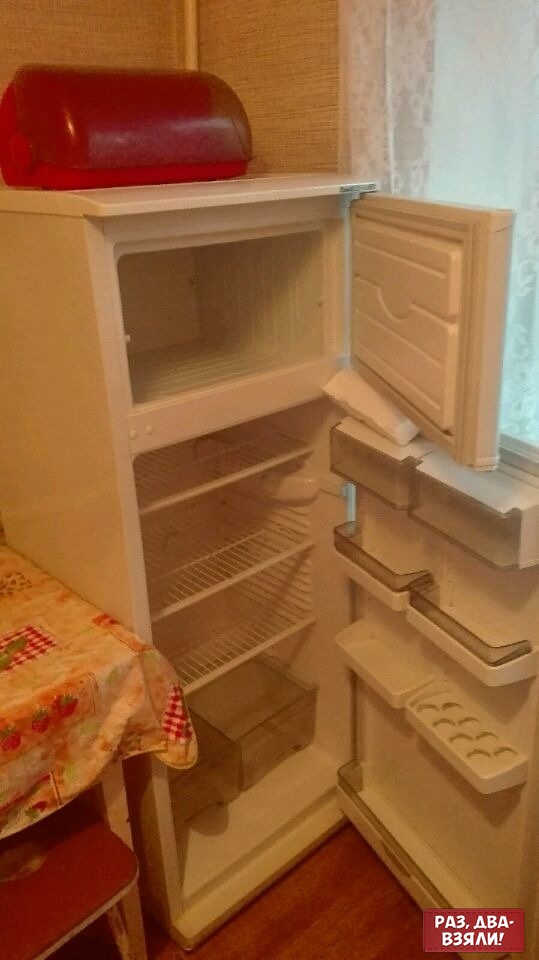This colored, somewhat vintage or filtered photograph depicts a small, white refrigerator with its doors open, revealing both an empty freezer on the top and an empty main cooler section on the bottom. The freezer appears to be defrosted. The fridge doors, which hinge on the right, obscure part of a window with a lace curtain that allows some bluish daylight to filter in. 

The kitchen walls feature a beige, woven-looking wallpaper, and to the left of the fridge, part of a dining table is visible. The table is adorned with a white tablecloth decorated with red, checkered patterns and strawberries, with a little red bench tucked underneath. A red, shiny plastic bread box or container sits on top of the refrigerator. The floors are a dark brown wood.

There is some text in the bottom right corner that includes "PA3" and "ABA," followed by non-English text and an exclamation point on a red background, which is unclear but seems notable in the context of the image.